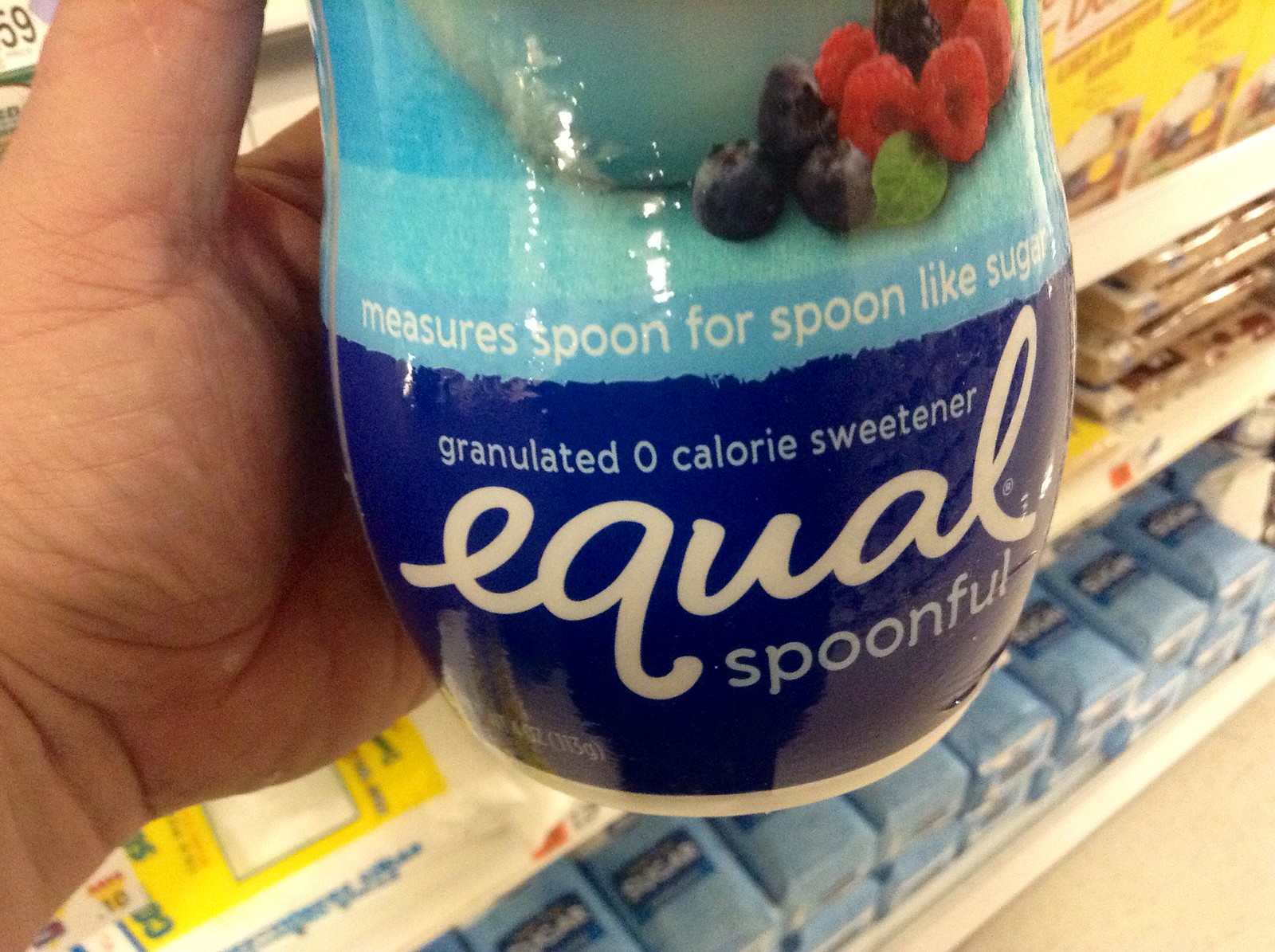In this detailed image, an individual is holding a plastic container of Equal's granulated zero-calorie sweetener, identifiable by its molded bottle with a shrink-wrap label that is predominantly light blue. The label features an image of a bowl filled with assorted berries, including blueberries, raspberries, and possibly a blackberry. Above the bowl, the text reads "Measure Spoon for Spoon Like Sugar" in white against a light blue background. Below this, the label transitions to a darker blue background with the text "Granulated Zero Calorie Sweetener" also in white. The brand name "Equal" is written in cursive, followed by the word "Spoonful" in a rounded typeface. The scene is set in a store aisle with a backdrop of shelves stocked with various types of sugars, including light brown sugar in boxes and bags, white sugar in blue paper bags, and bags of confectioner's sugar. The camera captures the image from about halfway down the container to the floor, emphasizing the hand holding the alternative sweetener against the sugary backdrop.